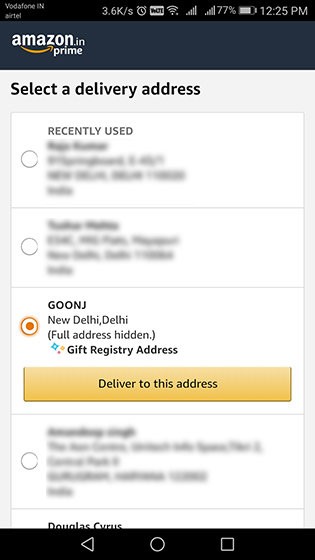**Caption:**

Vertical screenshot from a smartphone accessing the Amazon app or website. The topmost section has a black status bar displaying various indicators, including 'Vodafone in Airtel' on the left, data speed ('3.6K/S'), alarm clock icon, miscellaneous icon, Wi-Fi icon, and signal strength bars. The battery level reads 77%, with the current time being 12:25 PM.

Below the status bar, a dull black strip on the left corner reads 'Amazon.in' followed by the Prime logo. The interface allows the selection of a delivery address, displaying three options. The first two are blurred and not selected. The third option, which is selected, shows the address 'Goon J, New Delhi, Delhi (full address hidden)' and labels it as a 'Gift Registry Address' in bold. A yellow bar with black text below this reads 'Deliver to this address.' Another blurred, unselected address is partially visible underneath.

At the bottom, partial text hints at perhaps a user's name but is obscured by the black navigation bar featuring the triangle, circle, and square icons typical of Android devices.